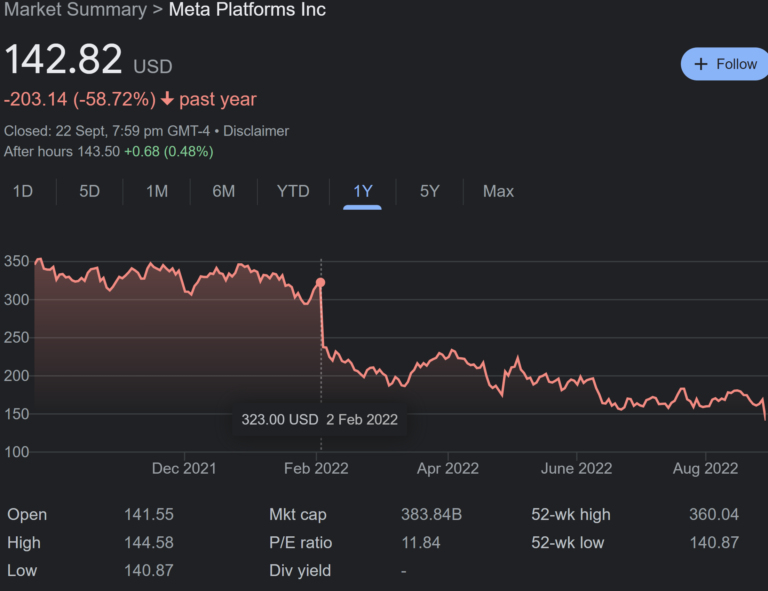### Detailed Caption for Financial Image:

The image primarily features a sleek black background with prominently displayed financial data. The centerpiece of the image is a white figure reading "142.82 USD," indicating a market summary for Meta Platforms, Inc. Below this figure, the words "Market Summary" are visible, followed by "Meta Platforms, Inc." in a smaller font, giving context to the numbers.

In the top right section, there's a blue oval button labeled "Follow" in black text, signifying an option to track or follow this financial instrument.

Highlighted in red, the image shows a significant negative figure: "-203.14" (in parentheses) along with a percentage of "-58.72%," indicating a substantial drop. Included alongside this is a downward arrow symbol.

Further to the right, there is a timestamp indicating the closing time as "22 SEPT, 7:59 PM GMT -4," and a disclaimer signifying after-hours trading data. The after-hours trading value is "143.50 USD" in green, showing an increase of "+0.68" or "0.48%."

A series of blue tabs labeled "1D, 5D, 1M, 6M, YTD, 1Y, 5Y, MAX" are displayed, likely offering various timeframes for observing the data trends. 

Beneath these tabs is a detailed chart, spanning from December 2021 to August 2022, with months abbreviated as DEC, FEB, APR, JUN, and AUG. Along the left axis, the chart is scaled in increments of 50, ranging from 100 to 350. Notably, as of December 2021, the chart line peaks at 320.

This comprehensive graphical display presents a clear and detailed overview of the financial performance and fluctuations of Meta Platforms, Inc. over the specified periods.